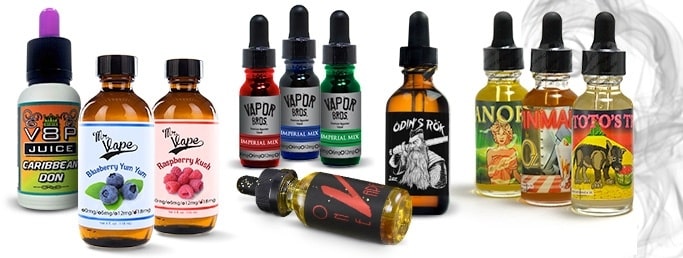This photograph, taken in portrait mode, showcases a diverse collection of small vape juice bottles, each adorned with distinct and colorful labels. On the far left, there are several fruity flavors including Mr. Vape Blueberry Yum Yum, featuring blueberries against a green background, and Mr. Vape Raspberry Kush, decorated with images of raspberries. Adjacent to these is V8P Juice Caribbean Dawn, notable for its purple tube and pink top. In the middle and towards the back, three solid-colored bottles from Vapor Bros stand in red, blue, and green, each marked with silver labels. At the front, a bottle labeled Odin’s Rock, illustrated with a Viking holding a sword, stands beside another tipped over bottle with a prominent red V. Over on the far right, a trio of bottles with artistic labels displays images such as a puppy and a woman, though the exact words remain unreadable. The setup and variety in the image suggest it might be an advertisement for vape juice flavors, highlighting the visual appeal of the product range.